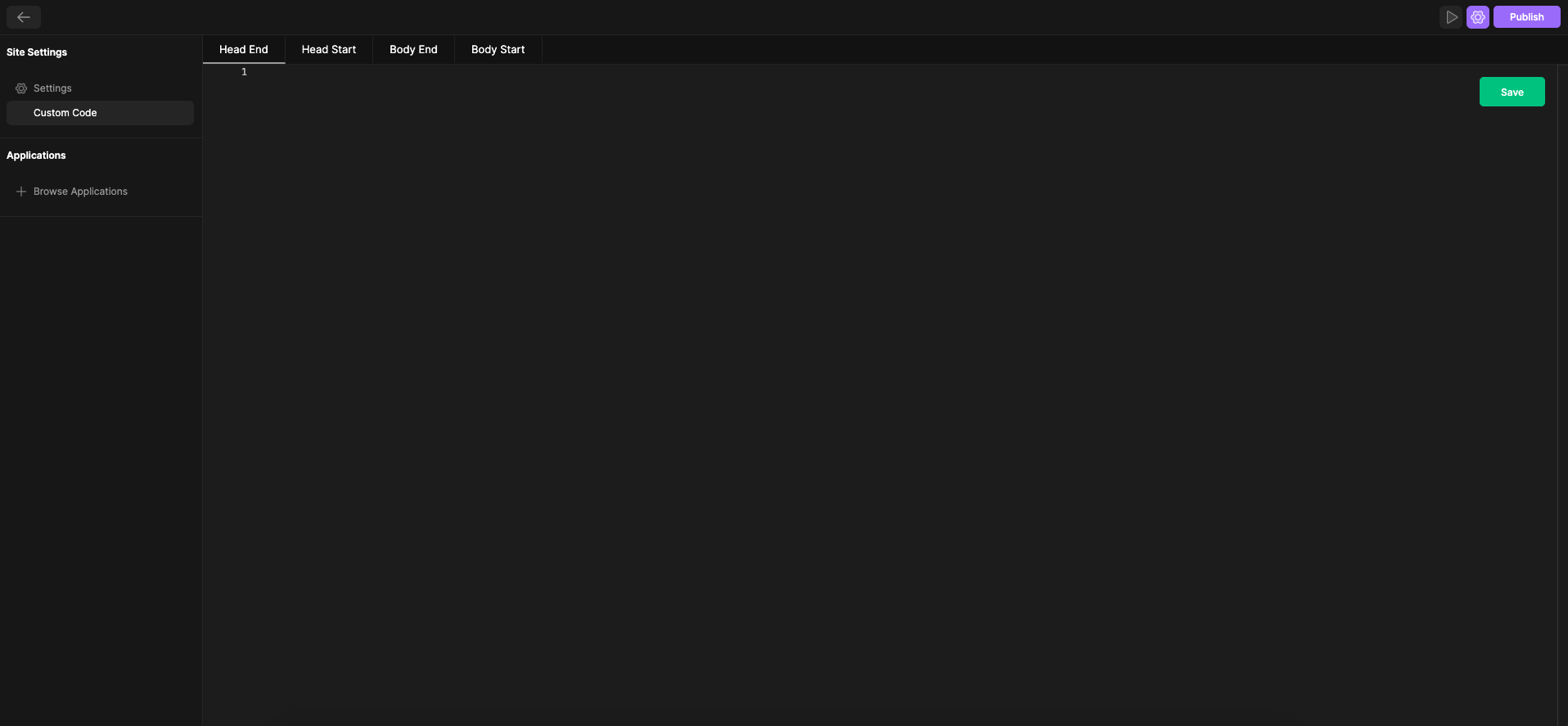The image appears to be a screenshot from a computer interface, displayed in a left-to-right horizontal orientation. The screenshot features a predominantly dark background with varying shades of black; a darker block is positioned along the upper ridge and down the left side, while a lighter, duller block occupies the middle section of the image. There is no observable texture or dimension within these blocks, but the difference in shading is noticeable.

In the upper left corner, there is a "go back" arrow icon. The upper right corner hosts an arrow icon pointing to the right, a purple settings icon, and a purple "Publish" button. Moving back to the left side of the interface, text elements appear: "Site Settings" in white, followed by a settings icon, and labels for "Custom Code" and "Applications" also in white. Below these labels, a gray button marked "Browse Applications" with a plus sign is visible.

Across the top of the screen are underlined labels in white: "Head End" with a small number one beneath it, "Head Start," "Body End," and "Body Start." Sliding over to the far right side of the screen, there is a small, rounded, green rectangular button with "Save" written on it in white letters.